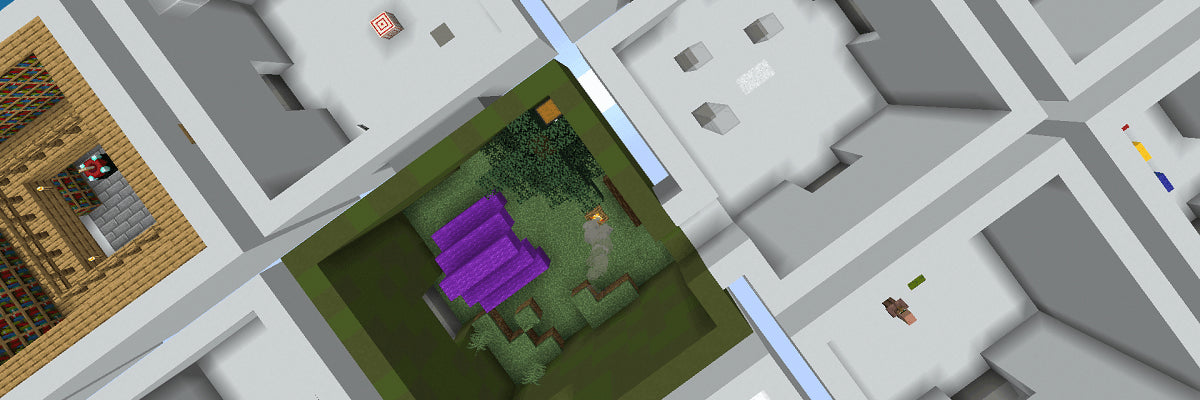This image, resembling a screenshot from a video game like Minecraft, provides an aerial perspective of a series of angular, cubicle-like rooms. To the far right, there is a distinctive brown room, possibly brick, featuring numerous smaller compartments and perhaps some bookshelves on the wall. Immediately adjacent is a prominently green room, filled with various green, Tetris-like shapes, and housing a notable purple staircase at its center. To the far left, a tan brick cubicle has a brown wooden floor, gray brick walls, and multiple holes in the floor, one of which is surrounded by a fence. This room also contains a red and white object, possibly a light, and another red and white box. Centrally, another room appears entirely green, with a purple staircase running through it, evoking a yard or garden-like environment. Scattered around these detailed rooms are several other cubicles, primarily white with gray walls and minimally furnished. These include a room with three boxes, one with a person standing in black and brown next to something green, and another additional cubicle on the far right with blue and green elements and red decorations.